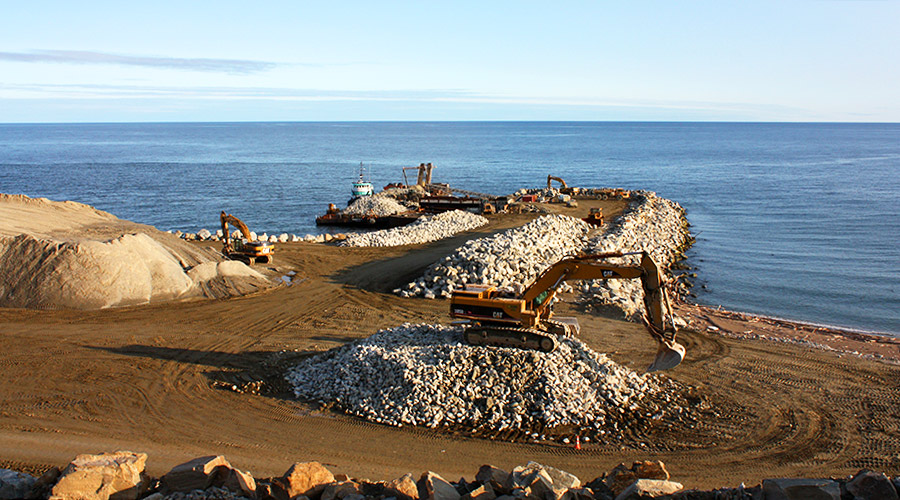This is a color photograph of a seashore construction site, likely a jetty under construction. Prominently, a yellow backhoe with the label "cap" on its side sits atop a raised mound of smaller rocks in the foreground. At the bottom of the image is a wall composed of large rocks. To the left of the main backhoe, next to a large mound of dirt, is another backhoe. The partially constructed jetty, made of rocks with a dirt road in the middle, extends out into the blue ocean, where another backhoe is visible at its end. Additional elements include a barge loaded with rocks, a white and blue tugboat alongside, and several mounds of rocks and sand scattered across the scene. The backdrop features the blue ocean meeting a white and blue somewhat cloudy sky. In summary, the detailed landscape features multiple excavators, large rock formations, equipment, and vessels, all contributing to the intensive construction activity along the shore.